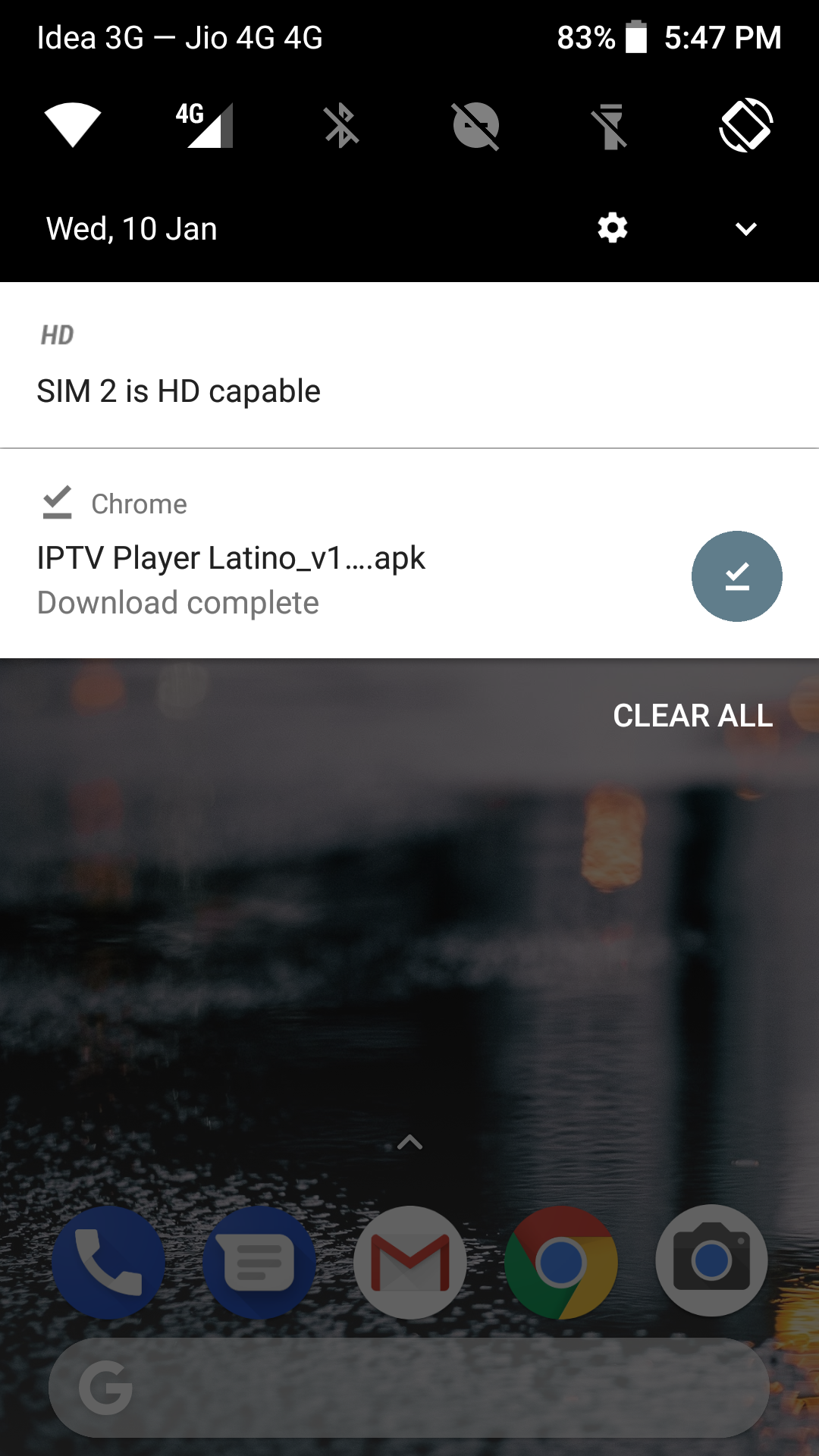In this image, the top left of the cell phone screen displays various status indicators: "IDEA 3G Geo 4G 4G" representing network connectivity, a battery life indicator at "83%,", and the current time "5:47 p.m". Beneath these indicators are six distinct icons: Wi-Fi, signal connection, Bluetooth, a Messaging icon with a diagonal line through it indicating it's disabled, a flashlight icon, and a rotate screen icon. Directly below, the date and day are displayed as "Wednesday, January 10th."

To the right of the date, there is a settings icon accompanied by a small downward arrow. Below this section is a notification stating "HD SIM 2 is HD capable," followed by another notification: "Chrome IPCV player Latino - v1.apk download complete" with a gray circle and a check mark. At the bottom part of the home screen, the text "Clear All" is displayed in white at the top right. 

The background of the home screen is a blurry image of what appears to be a faraway house, featuring gray and dark green shades. At the bottom of the screen, five app icons are neatly arranged: a call app, messaging app, mail app, Google Chrome, and a camera app. Below these, there's an oval-shaped button with a white uppercase "G" located at the bottom left corner.